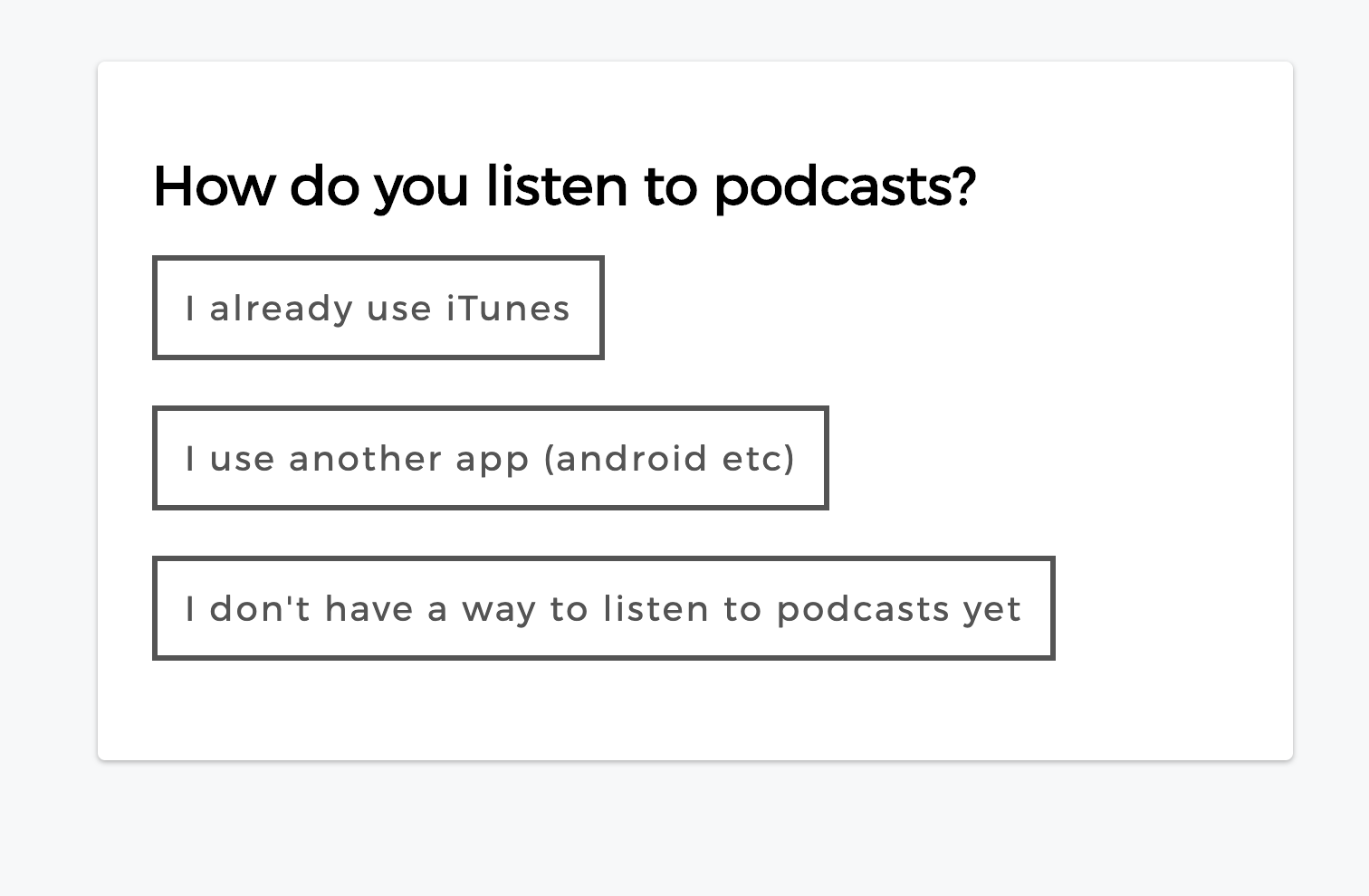The image displays a clean and minimalistic survey question form designed to assess podcast listening habits. The form features a light gray or white background, enhancing its simplicity and clarity. Enclosed within a rounded rectangular box adorned with a subtle shadow effect, the form stands out elegantly against the backdrop.

The title at the top of the form, "How do you listen to podcasts?" is prominently displayed in large, bold black text. The text is rendered in a modern sans serif font, ensuring readability and a contemporary aesthetic.

Beneath the title, three distinct options are presented as rectangular buttons, each bordered in gray with matching gray text. Ample spacing between the buttons clearly separates each choice:

1. "I already use iTunes": This button caters to respondents who use iTunes for their podcast listening needs.
2. "I use another app (Android, etc.)": This option is for individuals who utilize other applications or platforms on Android or other devices for podcast listening.
3. "I don't have a way to listen to podcasts yet": This choice addresses those who currently do not have any means to access podcasts.

The form’s layout is both functional and aesthetically pleasing, ensuring an intuitive user experience.